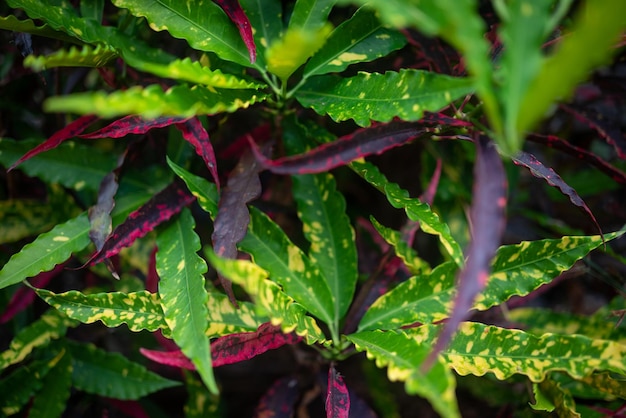This close-up photograph captures various leaves of a single plant species, showcasing a striking and diverse color palette. The leaves, predominantly long, narrow, and oval-shaped with pointed tips, fan out from short central stems, creating a clustered arrangement. The primary green leaves feature noticeable yellow spots or growths, with a varying density; some leaves bear only a few yellow marks, while others are more heavily spotted. Interspersed among the green leaves are deep purple leaves adorned with vibrant pink edges, adding to the plant's vivid appearance. Additionally, the lower section reveals more red and purple hues, creating a layered effect with both solid purple and red-spotted leaves. The intricacy and variety in leaf coloration and patterning are prominently highlighted in this detailed macro shot.